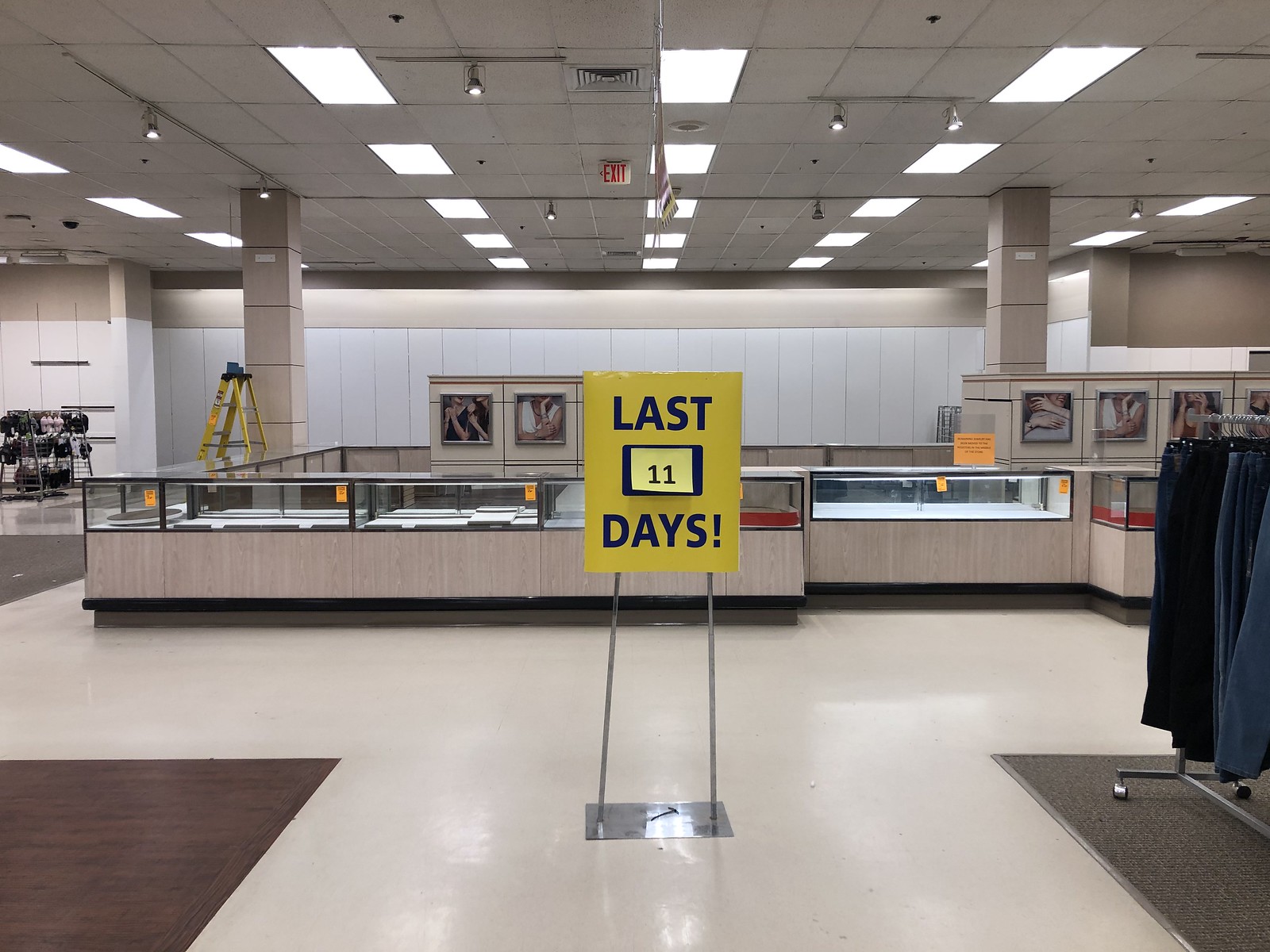The image depicts a department store in the midst of a going-out-of-business sale. The most prominent feature is a large, bright yellow sign that declares "Last 11 Days" in bold, attention-grabbing letters. Positioned directly behind this sign is a significant glass counter unit, which appears to be either a jewelry or fragrance counter. The counters are completely empty, making it difficult to ascertain their original purpose. Surrounding the counter area are various posters and promotional materials, though they are too distant to be legible or recognizable. To the right of the focal point, several racks of jeans are visible, neatly arranged. In the far left background, a rack displays a selection of shoes. The overall atmosphere is one of finality and clearance, marked by the stark emptiness and the visible reductions in inventory.